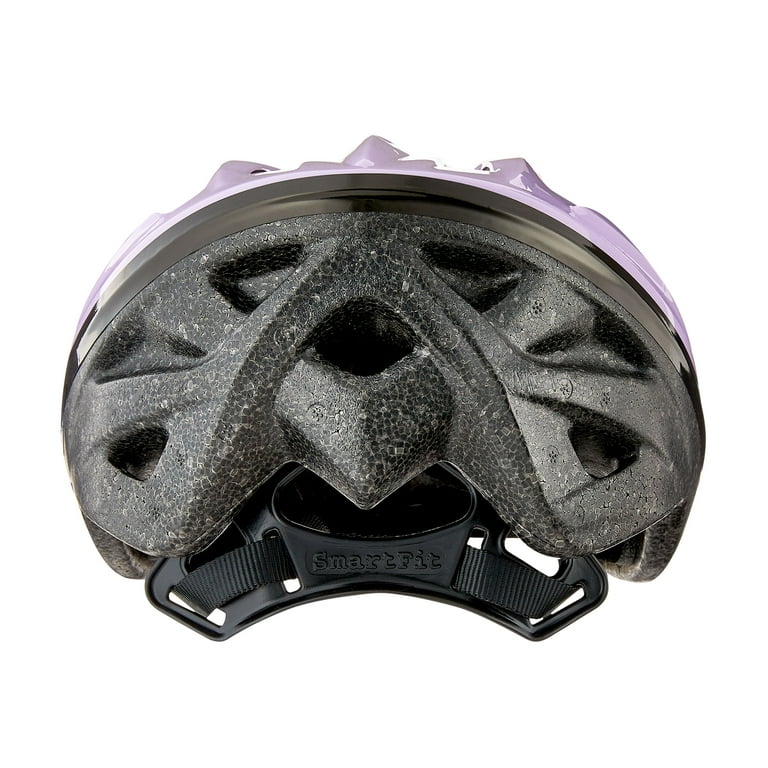This stock photograph showcases a bicycle helmet prominently against a white background. The visible section is primarily the back of the helmet, made of tightly compressed black styrofoam speckled with lighter gray, resembling a granite texture. Its design includes triangular indentations. You can also see a small portion of the top plastic exterior shell in a light lavender, lilac shade, with three point-like projections. At the bottom, the black rubber and nylon chin strap are visible, threaded through a black device likely used for display purposes in a shop. The helmet features a “smart fit” label in black, positioned around the area where the head and ear would rest, enhancing communication of the design and functionality of this protective gear.